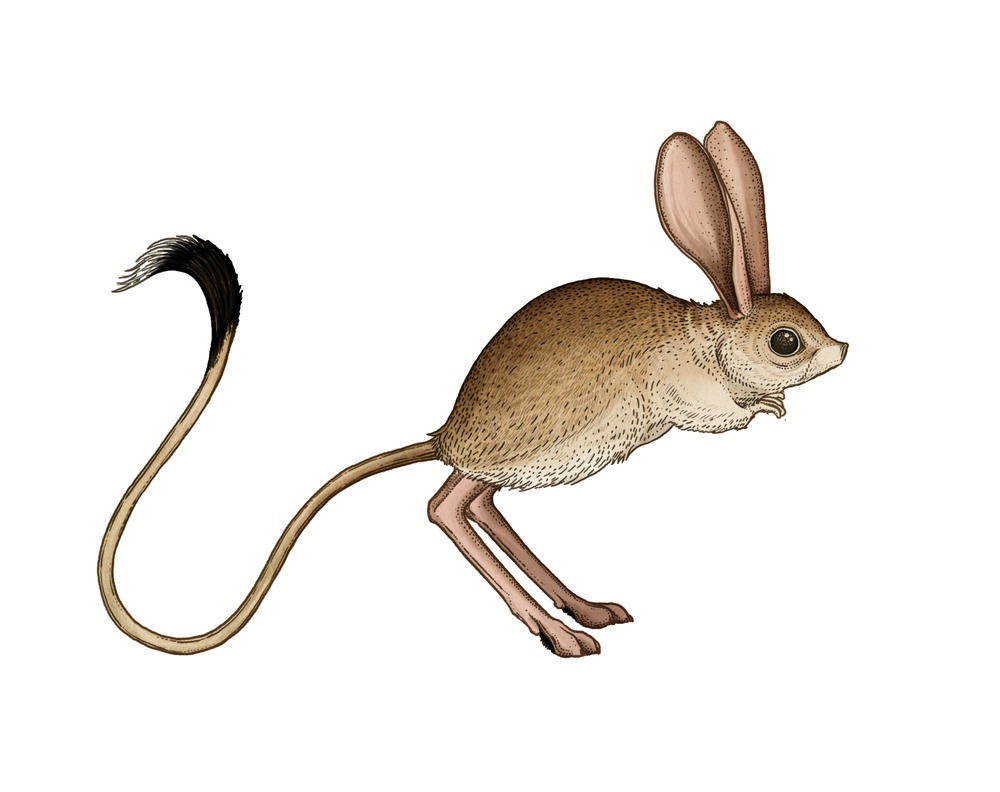The image displays a captivating, cartoon-like creature set against a completely white background. This unique animal, likely a type of rodent, features a blend of characteristics from various animals. It has incredibly long, bunny-like ears that stand out prominently. The creature's body is mouse-like, covered in brown fur with a darker tone on top and a lighter brown underbelly. Its expressive, doe-like eyes are large and bright, complemented by a tiny, pink nose. The front limbs are disproportionately tiny, reminiscent of T-Rex arms, while the hind legs are notably long, almost canine in appearance but lacking fur. A striking feature is its lengthy tail, which occupies about half of the total image space. The tail starts brown and transitions into a bushy, black-tipped end with a small touch of white at the very tip. Despite its unusual and varied features, the creature possesses a distinct charm and cuteness.